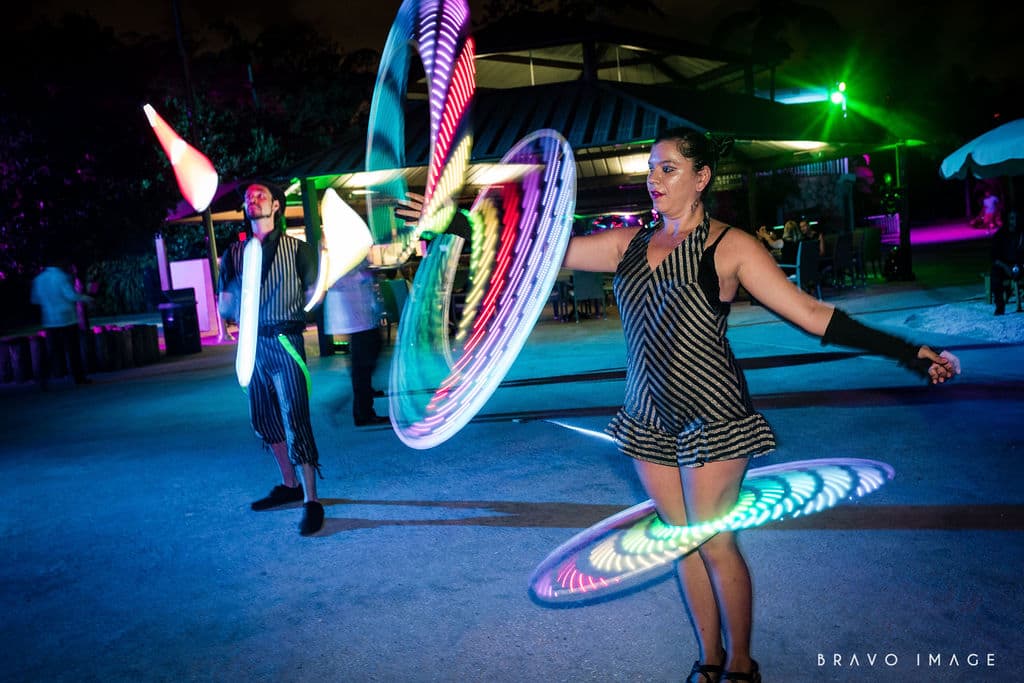This nighttime shot features two street performers impeccably clad in black and silver striped costumes. The woman sports a short romper with a halter neck and ruffled shorts, complemented by long fingerless gloves. She expertly spins lighted hula hoops—one mesmerizingly blurs around her upper knees while the other twirls rapidly in her hand, creating glowing rings of light. Beside her, a man in a loosely stylized suit and black shoes juggles illuminated clubs, their motion captured as three vibrant, blurry streaks. They perform on a concrete patio with a stage area and a few shadowy figures in the background. Overhead, a pavilion cover hints at a restaurant setting, with patrons seated at tables. In the bottom right corner, the words "Bravo Image" are subtly inscribed.